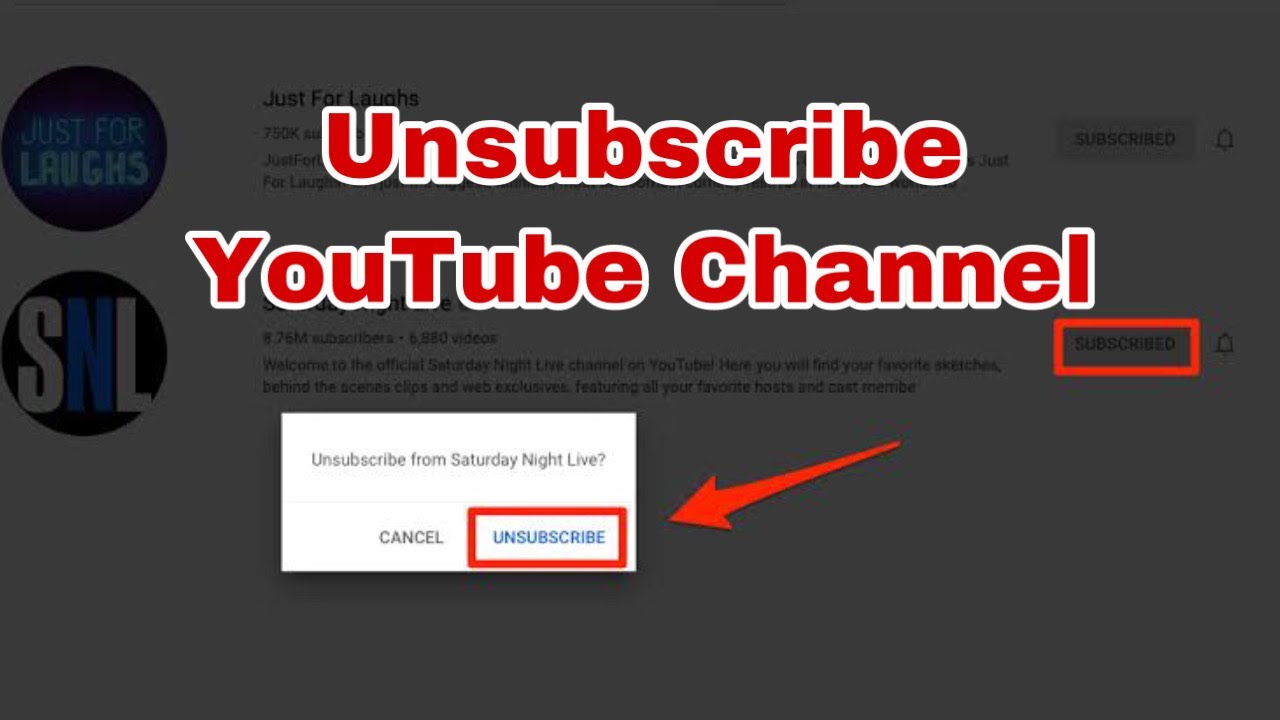The image displays a pop-up dialog box from YouTube with the title "Unsubscribe" prominently positioned within a red-bordered box. Beneath this title, there is a zoomed-in section emphasizing the word "Unsubscribe." Below this, there is a smaller block of text specifically stating "Unsubscribe from Saturday Night Live," indicating that the user is choosing to unsubscribe from the "Saturday Night Live" YouTube channel. The background slightly reveals another channel titled "Just for Laughs," though the primary focus remains on "Saturday Night Live." The dialog box features two options at the bottom: "Cancel" and "Unsubscribe," with "Unsubscribe" highlighted in the same red border as the title.